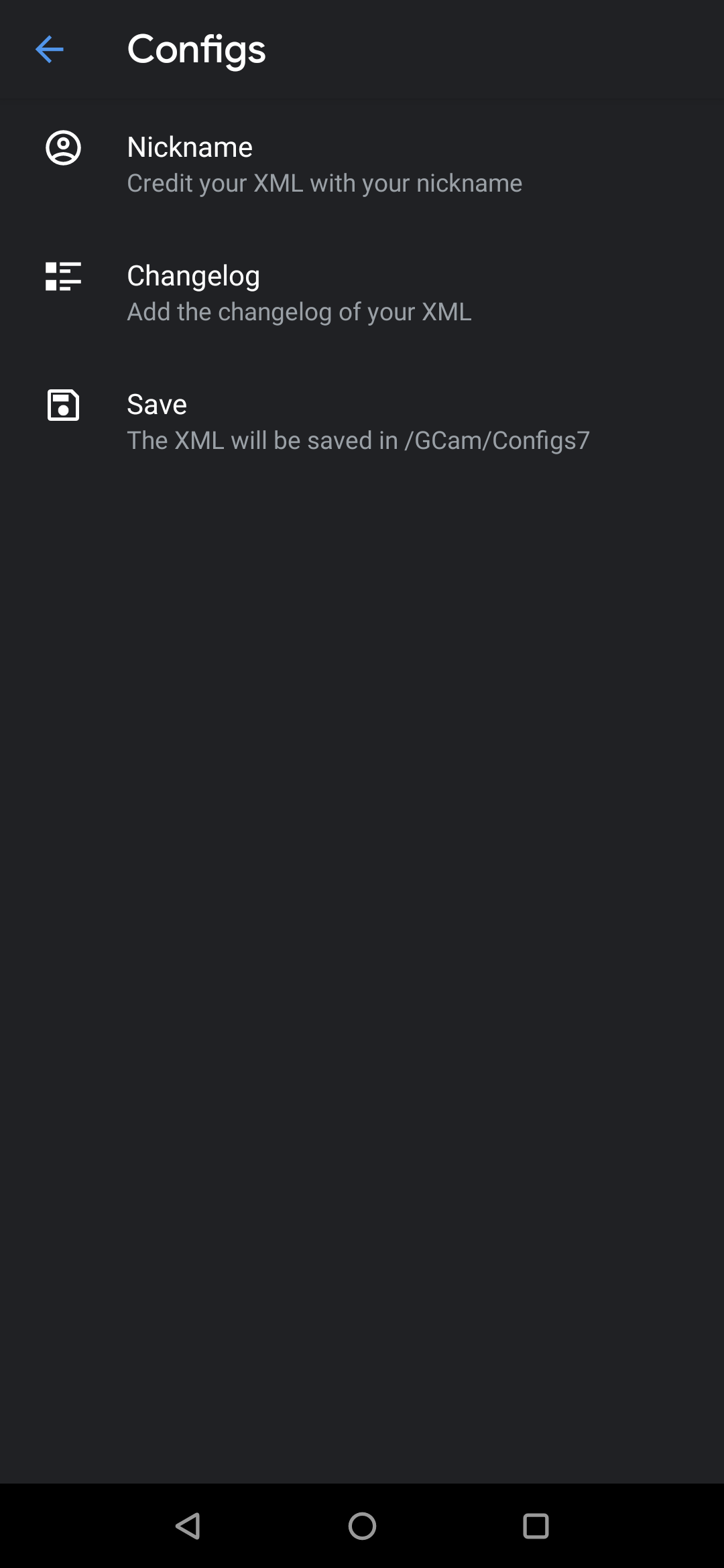This image is a screenshot from a cell phone app displaying a configuration screen. In the top left-hand corner, a blue arrow points to the left. To the right of the arrow, the word "CONFIGS" is prominently displayed in a large, white font. Below the title, a thin, dark grey line separates it from the main content of the screen, which consists of three categories.

The first category is "Nickname," accompanied by an icon depicting a person's head. The description reads, "Create your XML with your nickname." The second category is "Changelog," identified by an icon of two overlapping speech bubbles. Its description states, "Add the changelog of your XML." The third category, labeled "Save," features a floppy disk icon and the text, "The XML will be saved in /GCam/Configs7."

At the very bottom of the screen, the standard Android navigation buttons are visible: a back arrow on the left, a circular home button in the center, and a square icon on the right for accessing currently open applications.